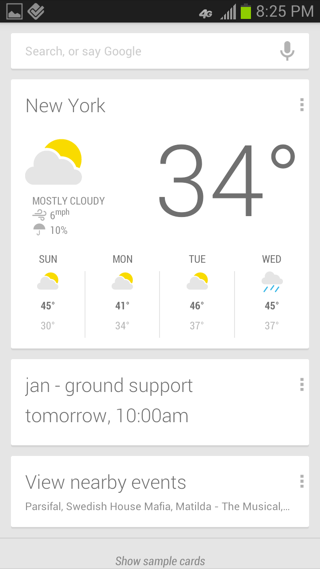The image displays a detailed weather forecast for New York City, alongside additional informational content. At the forefront is a search bar powered by Google, which is currently empty. The weather section prominently indicates that it is mostly cloudy with a brief appearance of the sun, and the current temperature is 34°F. The forecast from Sunday through Tuesday predicts similar weather conditions, while Wednesday is expected to bring rain. Specific temperature expectations are as follows: Sunday with a high of 45°F and a low of 30°F, Monday with a high of 41°F and a low of 34°F, Tuesday with a high of 46°F and a low of 37°F, and Wednesday with a high of 45°F and a low of 37°F.

Additionally, there is a notification about "Jan ground support" scheduled for tomorrow at 10 a.m. The section beneath advertises nearby events, listing "Paris Falls," "Swedish House Mafia," and "Matilda, the musical." Lastly, the image includes a prompt to "show sample cards."